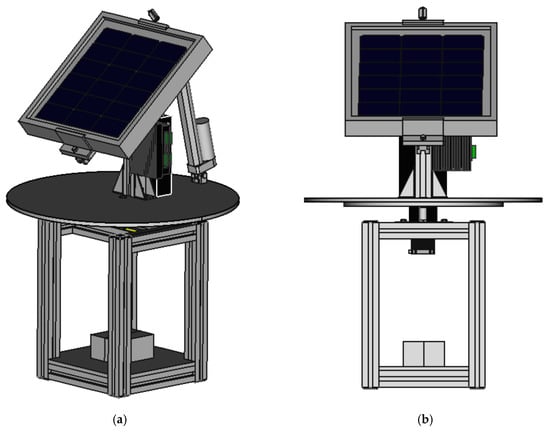This set of images labeled A and B displays a computerized, black-and-white generated photo of a single table and device from different angles. The table features a square base and a circular, black tabletop. Positioned on top of the table is a black stand supporting a square, adjustable box with a screen, possibly a monitor or drawing device, evident from its tiltable design. The box has two green buttons on the side, adding a touch of color to the monochromatic scene. The background in both images is white, emphasizing the grayscale palette of the table and device. Image A captures a side perspective, while Image B offers a frontal view, both illustrating the distinct black screen of the device held by an extendable arm. The entire setup suggests a modern, adaptable workspace or a specialized drawing station.